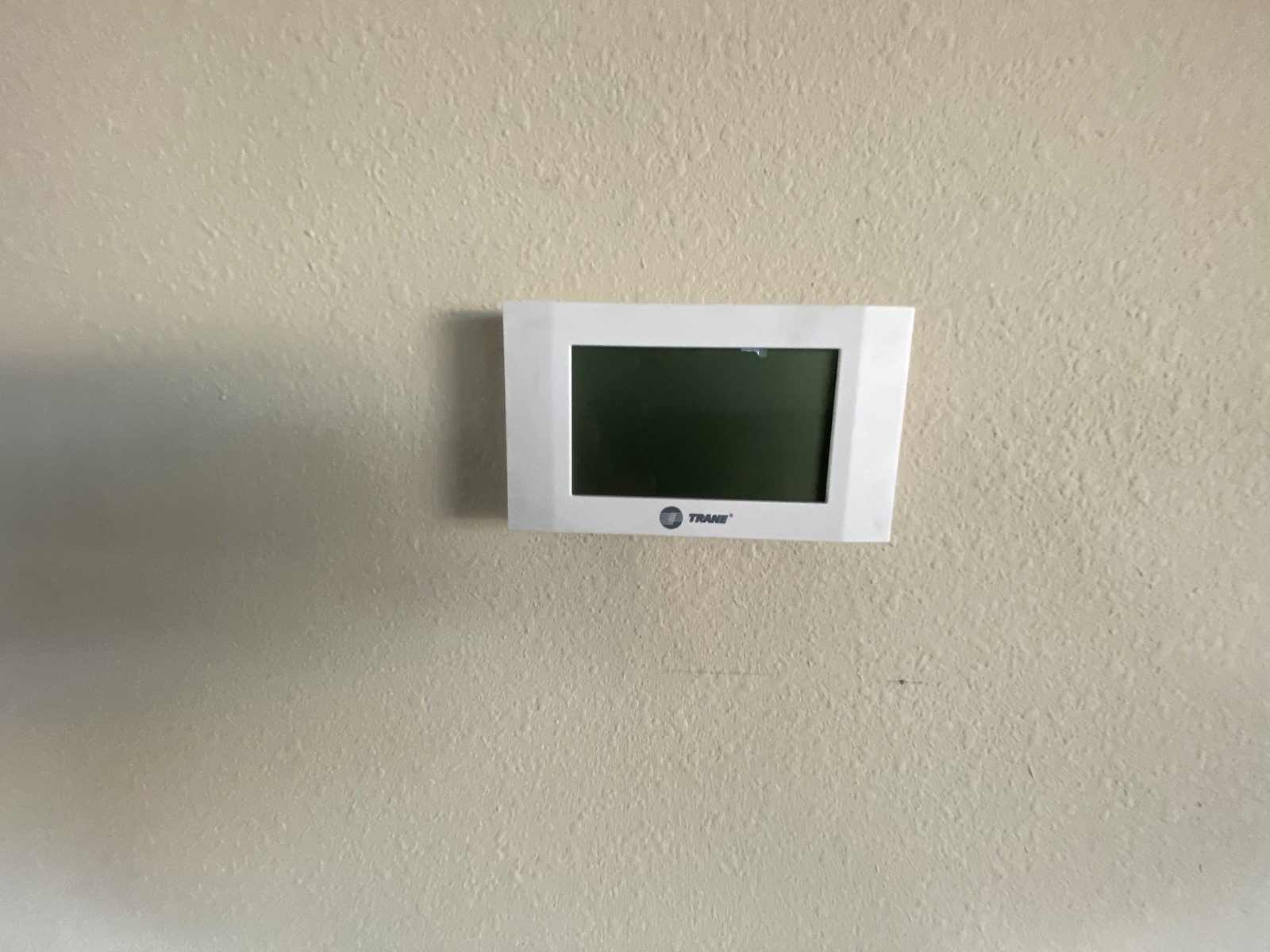The zoomed-in image features an off-white wall with a rough, bumpy texture. At the center, there is a bulky, rectangular electronic device that is also white. This device has a blank black screen in the middle, which is partially covered by a small piece of gray tape towards the top right corner. Below the black screen, there is a gray circle with white lines inside it. To the side of this circle is the bold, capitalized name "TRANE" in gray letters. Adjacent to the "E" in "TRANE," there is a small circle that might indicate a trademark or copyright symbol, but the details are unclear due to the zoom level.